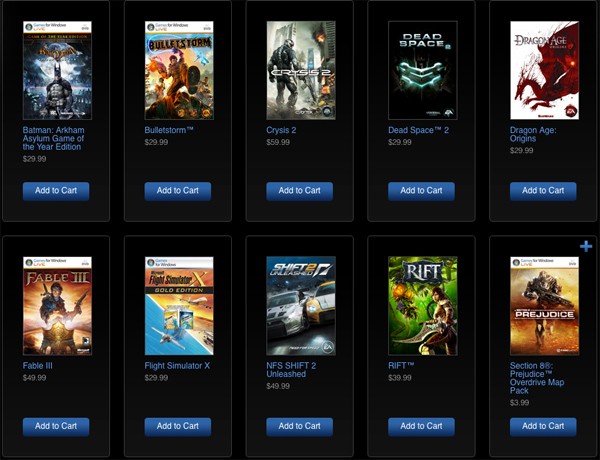This image showcases a collection of 10 video games available for sale, displayed in a 2-row arrangement with 5 games per row. 

Top Row:
1. **Batman** - Features cover art of Batman alongside an eagle-like figure.
2. **Bulletstorm** - Displayed next to the Batman game.
3. **Crysis 2** - Positioned alongside Bulletstorm.
4. **Dead Space 2** - Placed next in line.
5. **Dragon Age: Origins** - Occupies the final spot on the top row.

Bottom Row:
1. **Fable 3** - Marks the starting game of the bottom row.
2. **Flight Simulator** - Positioned next to Fable 3.
3. **Need for Speed: Shift 2 Unleashed** - Follows Flight Simulator.
4. **RIFT** - Positioned next in sequence.
5. **Prejudice** - Concludes the bottom row.

Each game is represented by its cover art, accompanied by a price tag ranging between $29.99 and $49.99. Below each price, a blue "Add to Cart" button with white text is featured. The entire display is set against a sleek black background, which highlights the vivid cover arts of each game.